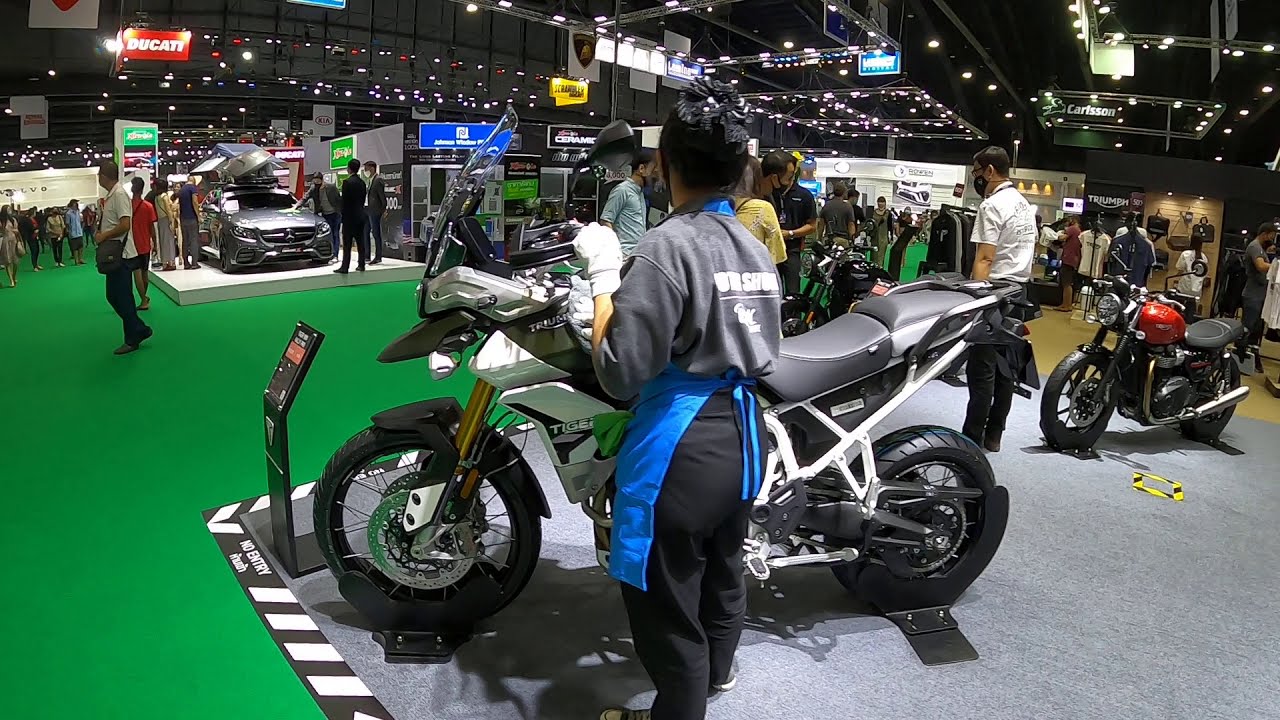This image captures an indoor auto and motorcycle convention set in a large, bustling exhibition hall with black ceilings illuminated by bright lights. Centrally positioned in the foreground is a prominent display of motorcycles, with three or four models visible, surrounded by a gray carpet area. Among the crowd, a man in a gray sweatshirt, blue apron, and black pants, potentially cleaning or inspecting a motorcycle, stands out. To the side, a sleek, gray Mercedes car is also on display, set against a white carpet floor. The surrounding area features a green carpet, adding a splash of color to the scene. Numerous visitors are seen milling about, engaging with the exhibits. Hanging overhead on the left side, a red sign with white lettering reads "Ducati," hinting at the prestigious brand of some of the displayed motorcycles. Various informational signs and indicators point towards other high-end car brands, including Bugatti, enhancing the convention's upscale ambiance. The overall setting is lively and well-lit, creating a stark contrast with the dark exterior visible through some sections.